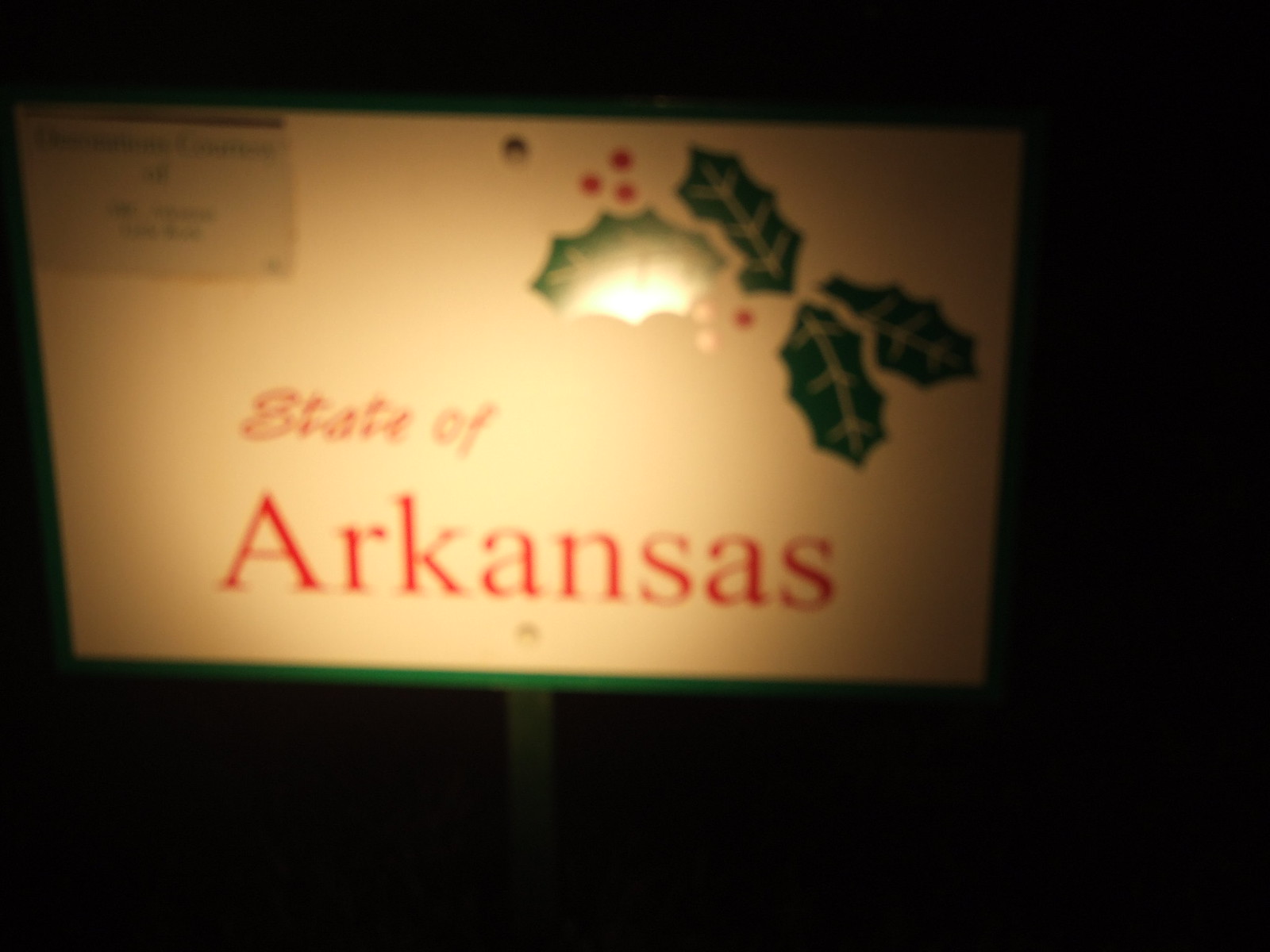A slightly blurred color photograph depicting a sign for the state of Arkansas, taken at night with a flash, resulting in a stark black background. The sign is mounted on a metal pole that extends downward to the bottom of the image. Prominent red letters spell out "Arkansas" in a large font, positioned against a primarily white or beige backdrop with a green border framing the sign. In the top right corner, there is a decorative design featuring green holly leaves and red berries. The sign also includes a small card-shaped area in the top left corner that contains some text, although the details are indiscernible.